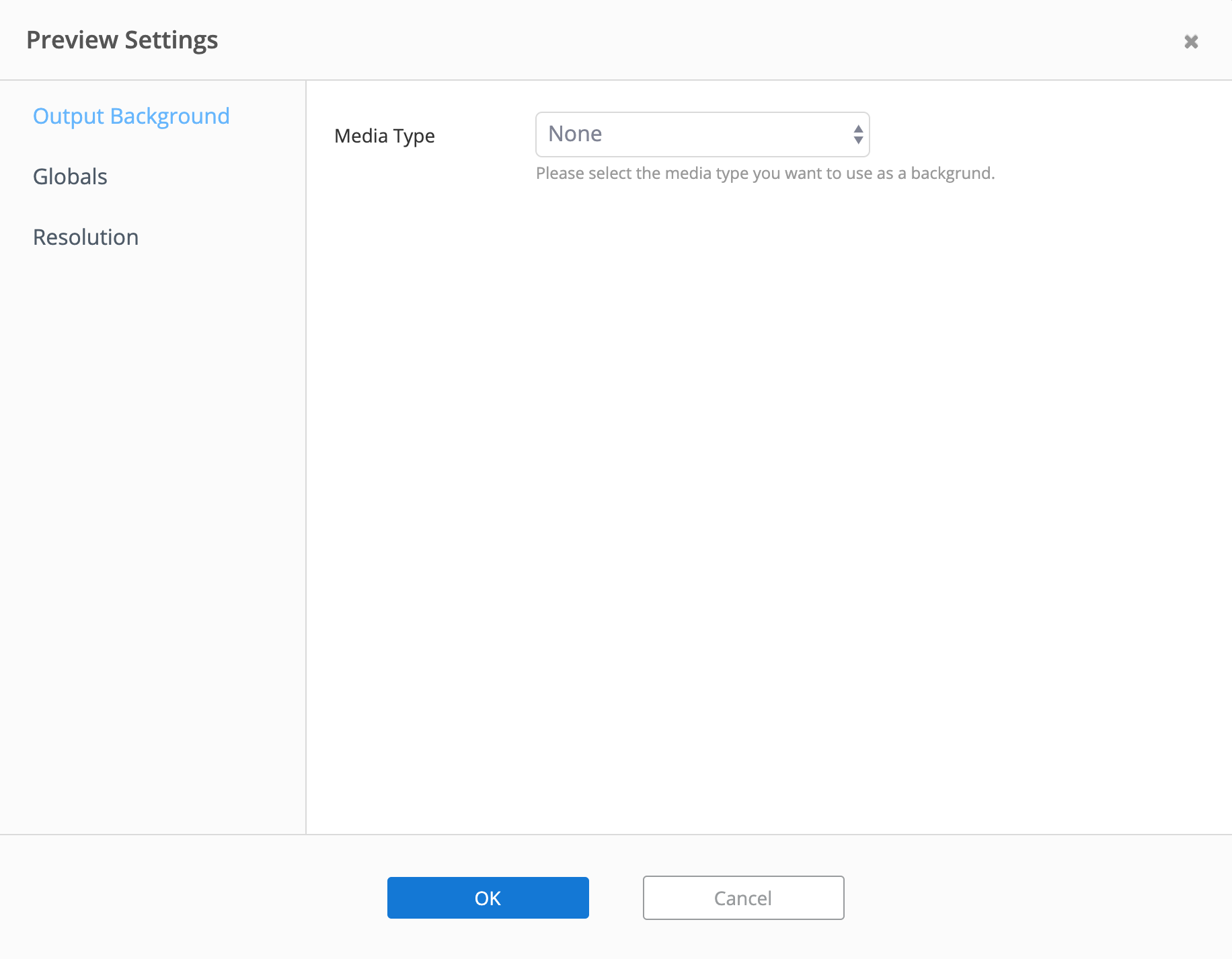The image features a user interface with a light gray border that runs along the top, left column, and bottom edges. This border is delineated by a slightly darker gray line, creating a boxed-in effect for both the left column and the top banner. 

The top banner, labeled "Preview Settings," is situated within this border and includes a black "X" icon on the right side for closing the settings. 

The left column is divided into three sections, the first of which is marked by blue text that reads "Output Background." This section appears to be selected, while below it, in black text, are the options "Globals" and "Resolution."

Moving to the primary middle section of the interface, it features a clean white background. On the top left of this section, the text "Media Type" is displayed. Directly beneath this, there is an outlined white box containing the word "None," accompanied by a toggle switch on the right. This area is annotated with the instruction, "Please select the media type you want to use as a background."

The overall design is minimalistic, focusing primarily on these interface options without additional extraneous elements.